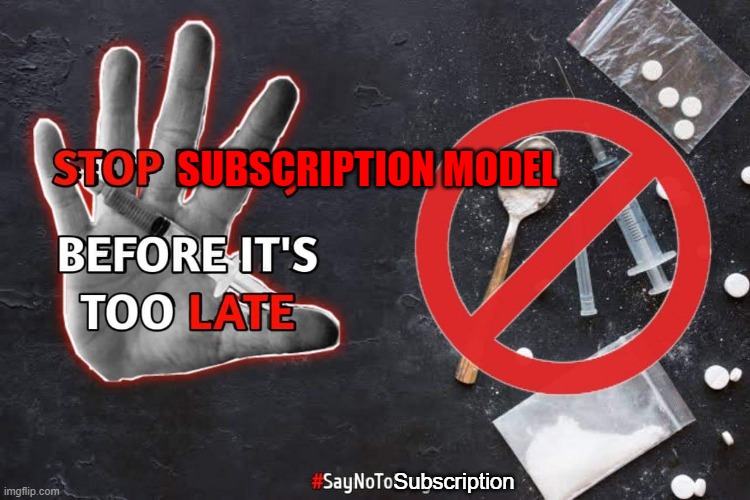This black and white image features a disembodied hand on the left, predominantly in gray and black tones, with vivid red text on it reading "Stop Subscription Model" and "Before it's too late," where "late" is also highlighted in red. The hand floats mysteriously, missing its wrist and arm. On the right side of the image, various drug paraphernalia including a spoon with a wooden handle coated in white powder, a large and small syringe, and scattered pills are partially obscured by a "no drugs" symbol—a circle with a diagonal line through it. In total, there are thirteen pills: four in a plastic bag, four next to the stop symbol, one inside the symbol, and four circular ones standing on end. At the bottom center of the image, bold red text framed by a red hashtag reads "Say No to Subscription," with significant letters capitalized. The lower left corner bears the watermark "imgflip.com," indicating the source of the image. The entire scene is depicted as if it were laid out on a dark, textured road surface, enhancing the stark and gritty mood of the image.